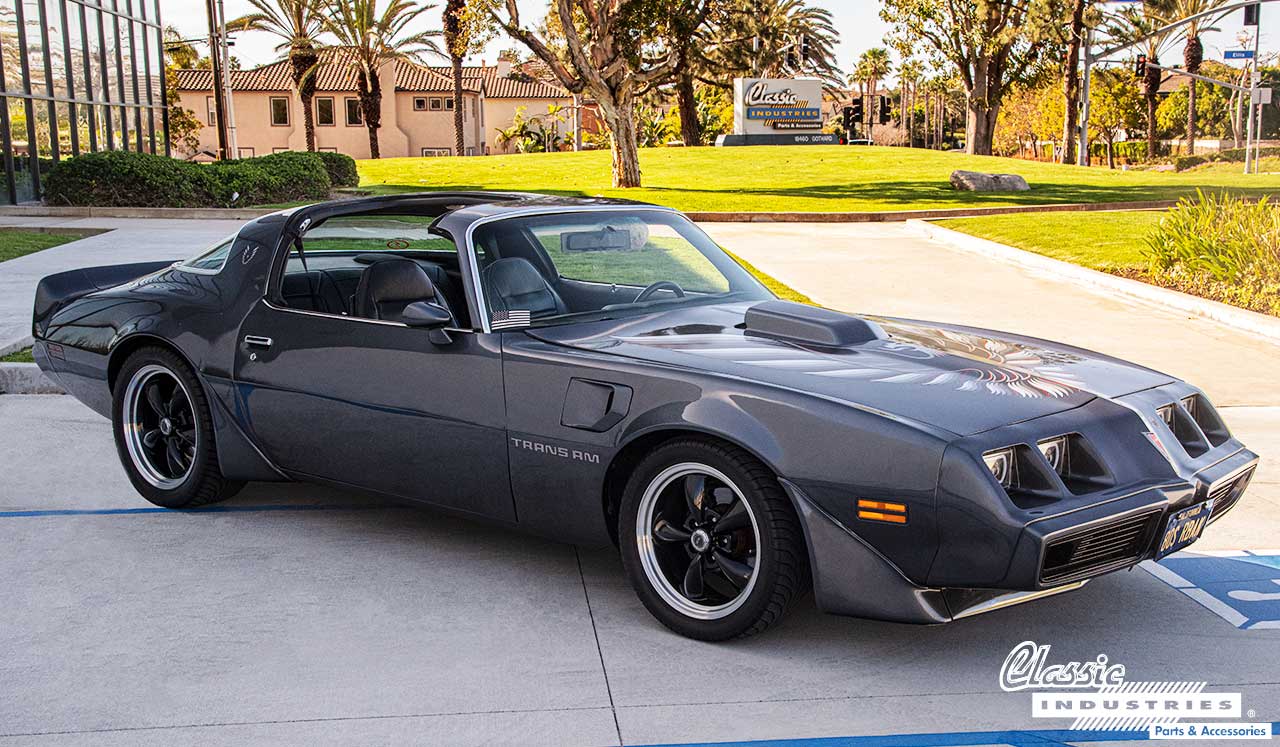This photograph captures a detailed side-profile view of a striking black Trans Am sports car from the 80s, parked on a large light-gray cement surface. This iconic vehicle, adorned with T-top convertible features and a distinctive angular old-school body style, showcases a glossy black paint job and custom tires with black rims encircled by a silver outline. The front end of the car reveals four square headlights and a hood adorned with an artwork that resembles a winged creature, accompanied by a hood vent. The car’s side clearly displays the "Trans AM" emblem in bold letters, evoking a sense of nostalgia and performance. 

Positioned in what appears to be a spacious parking lot on a sunny day, the background includes vibrant greenery, several palm and other trees, a pink building to the left, and California-style houses under a sunny sky, suggesting a location in California. An American flag drapes the passenger side of the windshield, enhancing the classic Americana vibe. Prominently visible, both at the bottom right and in the background, is signage for "Classic Industries Parts and Accessories," implying that the car serves as an advertisement showcasing their restoration capabilities. The entire setting portrays a picturesque and meticulously maintained classic car, elegantly poised to highlight its heritage and charm.